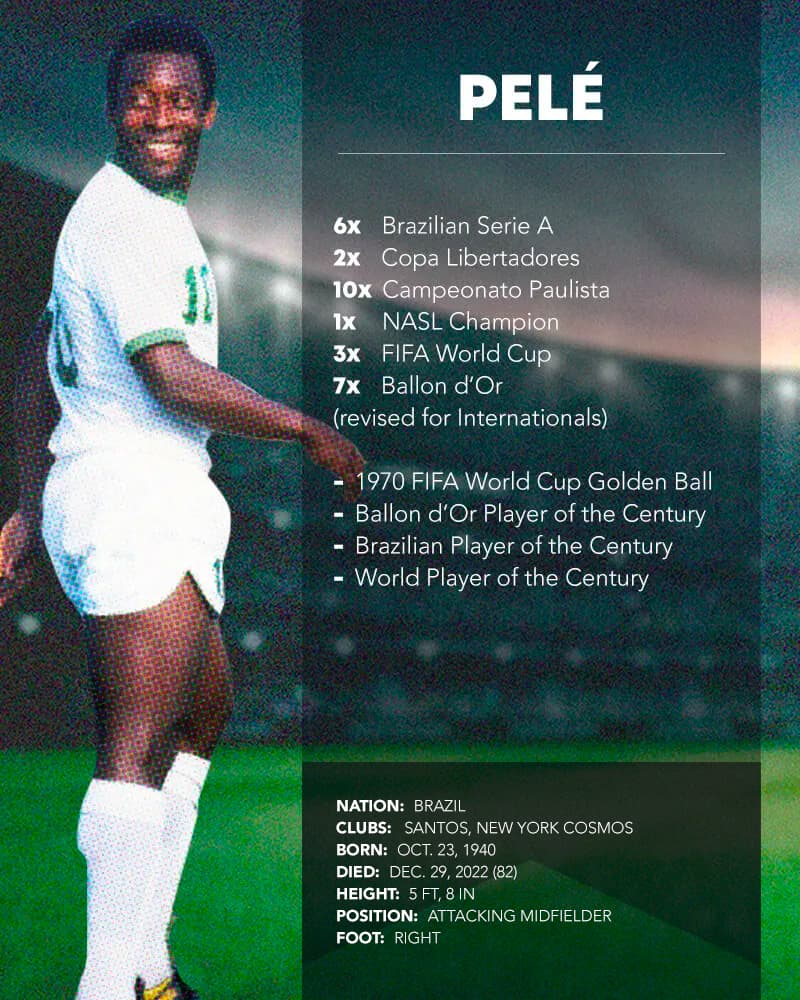This captivating poster features the renowned soccer star Pelé, presented with a photograph of Pelé on the left-hand side, adorned in a white soccer suit with green edges and numbers. He stands against a faded background of a soccer field, signifying his illustrious career. On the right-hand side, set against a dark, transparent rectangle, is an extensive biography detailing his monumental achievements in white text. The text celebrates his numerous accolades: 6x Brazilian Serie A champion, 2x Copa Libertadores winner, 10x Campeonato Paulista titleholder, 1x NASL Champion, 3x FIFA World Cup victor, and 7x Ballon d'Or (Revised for Internationals). It also highlights his awards such as the 1970 FIFA World Cup Golden Ball and titles like Ballon d'Or Player of the Century, Brazilian Player of the Century, and World Player of the Century.

Further details provide an overview of his legacy: his nationality (Brazil), affiliated clubs (Santos and New York Cosmos), birth date (October 23, 1940), and death date (December 29, 2022) at the age of 82. Additional statistics note his height (5 feet 8 inches), playing position (attacking midfielder), and primary foot (right). This comprehensive poster not only honors his achievements but also offers a complete portrait of one of soccer’s most legendary figures.